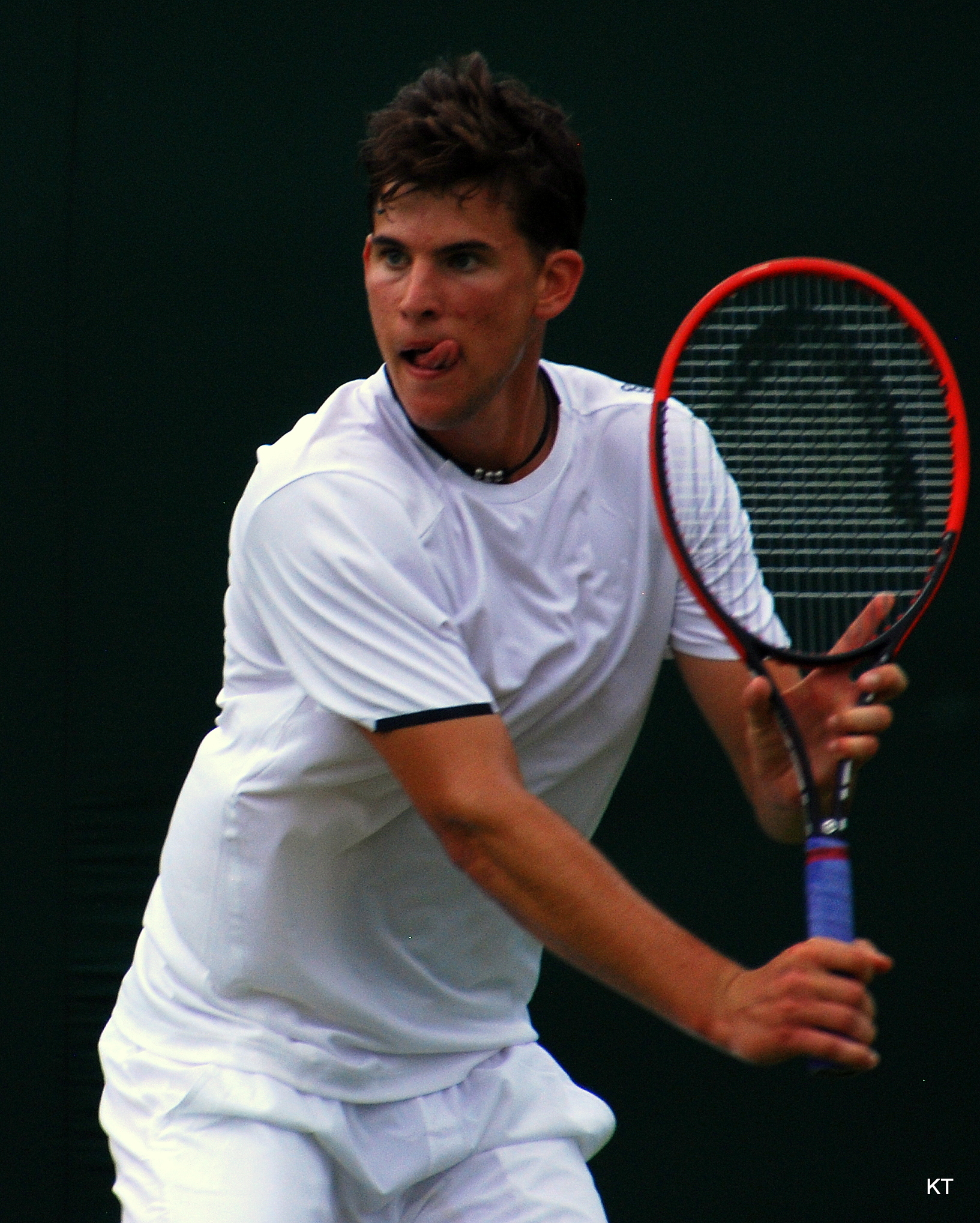The image captures a young male tennis player in his 20s, exuding determination and intensity. The background is black, making the subject stand out prominently. He sports a white short-sleeve t-shirt accented with black around the arms and a pair of white shorts. His hair is short but thick, with some strands falling onto his forehead, dampened by sweat. His dark eyebrows and eyes contrast sharply against his fair complexion, which is flushed from exertion. Perspiration glistens on his face as he sticks his tongue out, seemingly to lick sweat off his upper lip. Around his neck is a distinctive black necklace adorned with three silver balls. The player holds a tennis racket with a blue handle and a red top, poised in anticipation of the next move. The racket features a black frame with red trimming around its circular head. His serious expression suggests focus and readiness for the incoming ball. In the bottom right corner of the image, the initials “K” and “T” are displayed in white text.